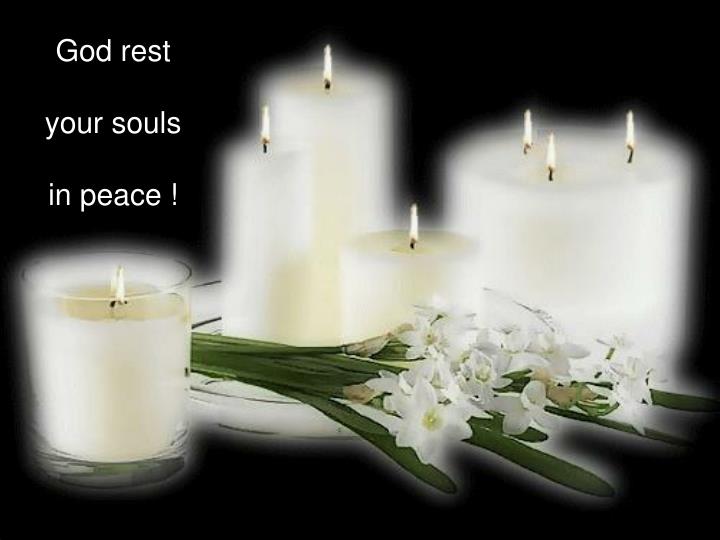This rectangular image, approximately nine inches wide by seven inches tall, is a serene and solemn digital creation, often used to express condolences for a recent loss or commemorate a group historically honored on specific days. Set against a stark black background, the scene is softly blurred to invoke a heavenly halo effect. It prominently features five candles of different shapes and sizes, with all of their wicks lit. On the left, a single white candle is encased in glass, while the center displays three candles of varying heights placed together on a shallow glass dish. Another large three-wick candle stands on the far right, casting an even, gentle light. Across the image, some white daffodils—possibly mistaken for lilies—are draped lightly, adding a touch of delicate floral grace. In the upper left corner, a poignant message in white text reads, "God rest your souls in peace!" capturing the essence of mourning and remembrance.